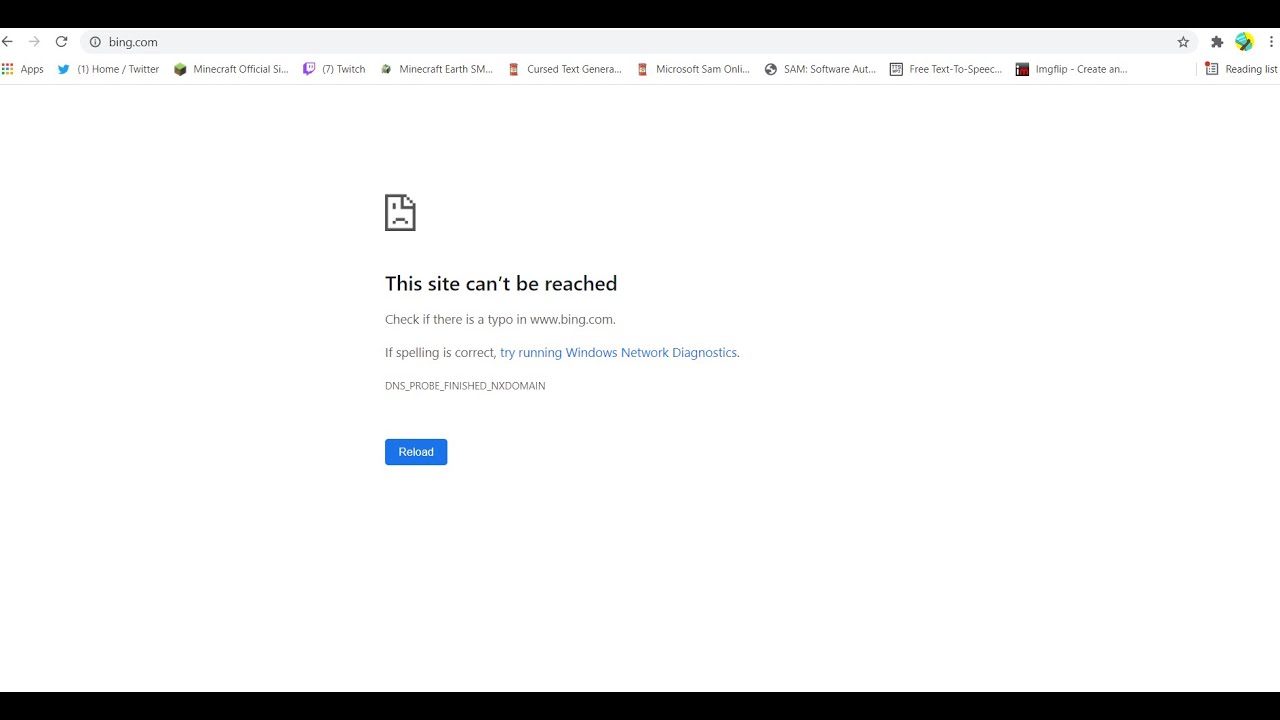This image is a screenshot of a web browser displaying an error message indicating that the site could not be reached. The URL bar at the top shows that the user attempted to navigate to "www.bing.com." Below the URL bar, there is a row of pinned icon shortcuts, approximately 10 in total. These shortcuts include commonly used sites and apps such as Twitter, Minecraft Official, Twitch, Minecraft Earth SM, Cursed Text Generator, Microsoft, SAM, 5AM Software, Free Text-to-Speech, and Image Flip. On the left side of the screen, there is a label that reads "Apps." Prominently featured in the center of the screen is the error message "This site can't be reached," with a suggestion to check if there is a typo in "www.bing.com." The overall layout highlights the browser's interface and the specific network error encountered.